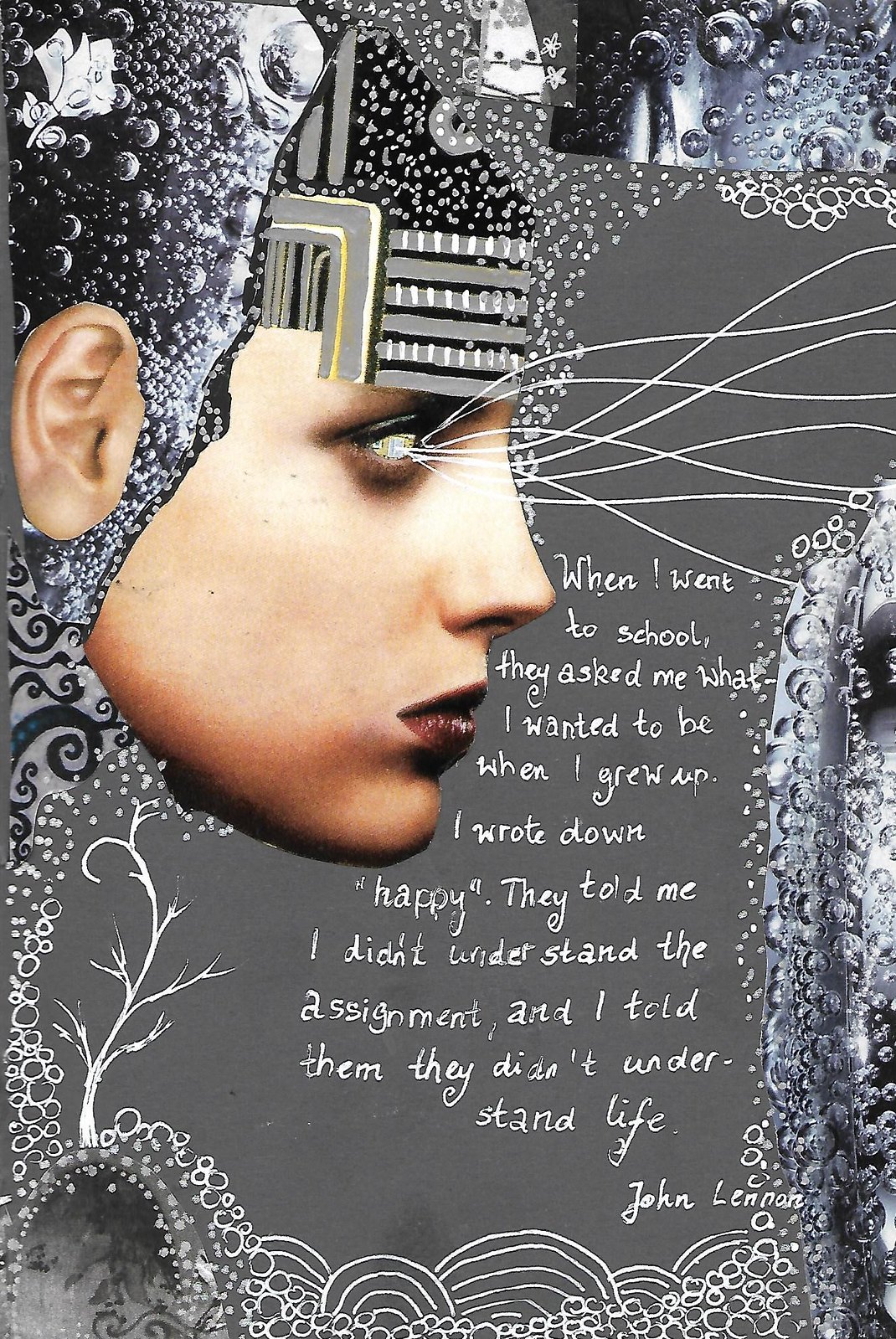The image is an abstract, rectangular artwork predominantly painted in shades of gray. It features a collage-style composition that is taller than it is wide. The focal point of the piece is a female Caucasian head located in the upper left corner, positioned in profile and facing to the right. Her face seems to emerge from a sea of gray bubbles that frame the image's border and cascade down the right side. The woman has red lipstick, a robotic-looking forehead, and empty white eyes from which silver, thread-like streamers extend toward the right side of the artwork. 

In the bottom left corner, the bubbles and gray background give way to an intricate white image resembling a bald tree, evoking elements of nature such as hills and valleys. 

Central to the composition is a handwritten quote in white text, placed to the right of the woman's nose and descending vertically. The text reads: "When I went to school, they asked me what I wanted to be when I grew up. I wrote down 'happy'. They told me I didn't understand the assignment, and I told them they didn't understand life." The quote is attributed to John Lennon.